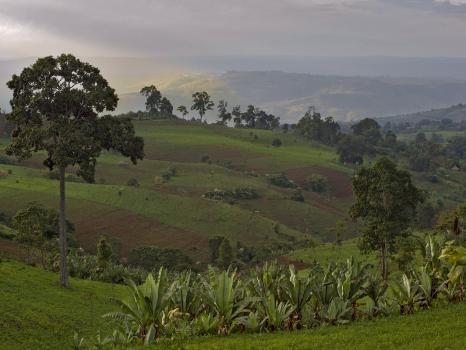This photo, taken in the countryside, captures a vast, lush landscape of rolling green hills extending across the frame. The foreground features an array of yucca-type plants with large leaves sticking up and slightly falling to the side, all set against a backdrop of short, dark green grass. In the midsection of the image, a scattering of trees continues along the hills as they roll off to the right. A single, thin-trunked, deciduous tree stands tall on the left side, its rounded, leafy top reaching about 30 feet high. The distant hills appear hazy, accentuated by a light gray, overcast sky that brightens slightly in the top left corner. No animals or people disrupt the serene, expansive landscape.